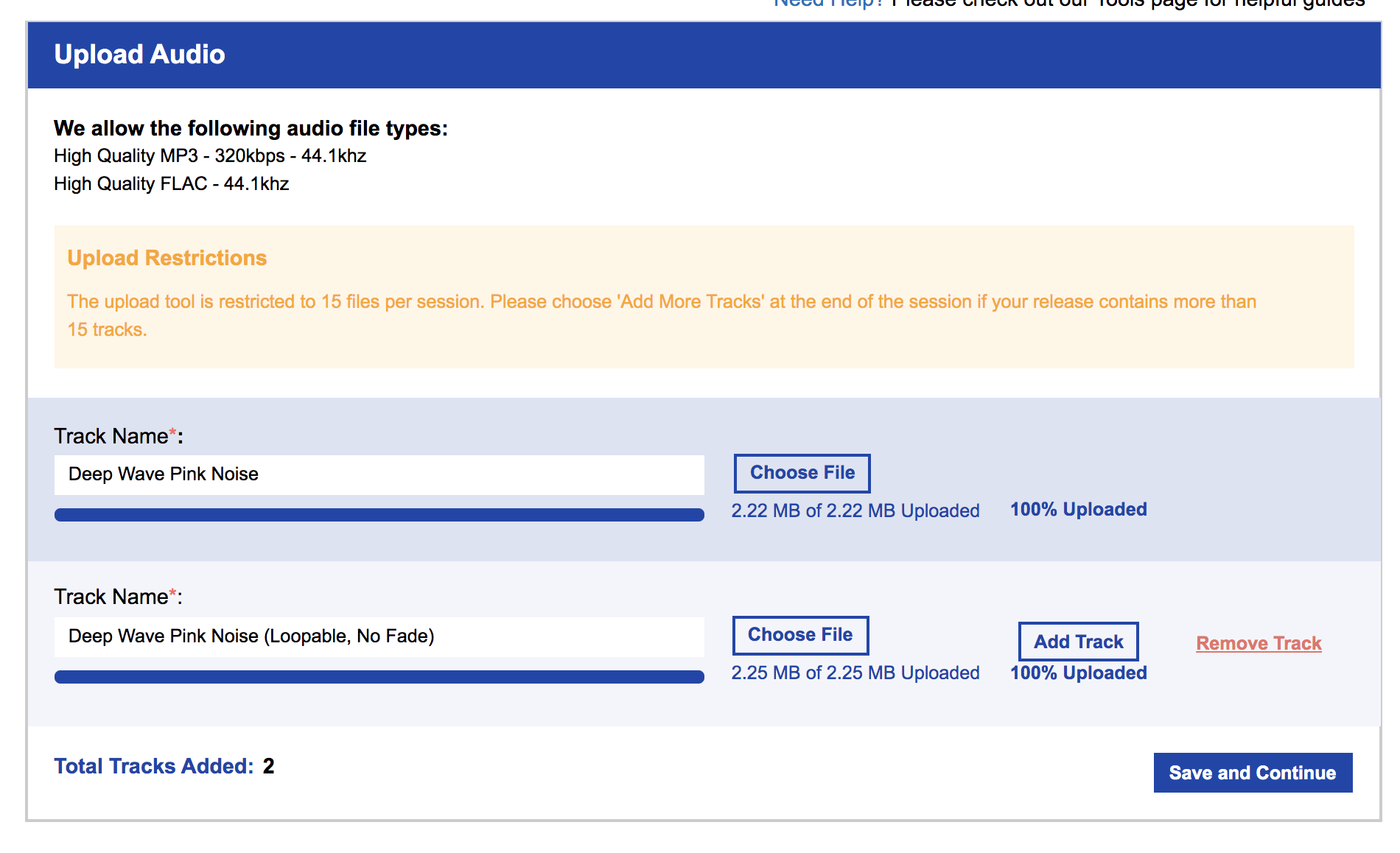A detailed view of an audio upload interface is depicted. At the top of the screen, a blue bar prominently displays the text "Upload Audio." Directly below, the interface outlines acceptable file formats with the message, "We allow the following audio files: high quality MP3-320KBPS-44.1KHZ and high quality FLAC-44.1KHZ."

An orange bar follows, highlighting upload restrictions: "Upload Restrictions: The upload tool is restricted to 15 files per session. Please choose Add More Tracks at the end of the session if your release contains more than 15 tracks."

Beneath this is another blue bar indicating the first track's name, "Track Name: Deep Wave Pink Noise," with a status bar below it indicating file upload completion: "2.22 MB of 2.22 MB uploaded, 100% uploaded." 

The next segment shows the second track labeled, "Track Name: Deep Wave Pink Noise, Loopable, No Fade," also with a blue status bar and an upload indicator: "2.25 MB of 2.25 MB uploaded, 100% uploaded." 

Options to add or remove tracks are available, and at the bottom, a summary states, "Total Tracks Added: 2." The screen concludes with a "Save and Continue" button, indicating the next possible step in the upload process.